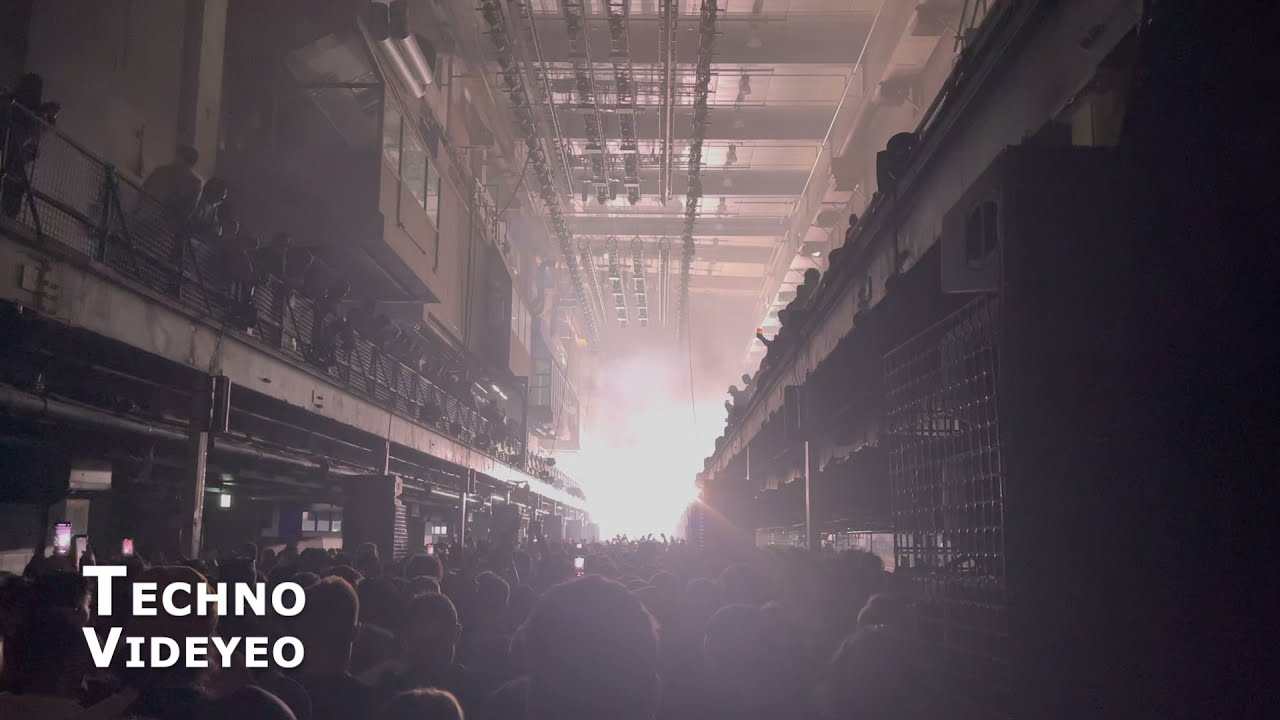The image appears to capture a dark, sepia-toned photograph of what seems to be an impromptu rave inside a commercial, industrial building. The structure features a metal roof and exhibits an overall industrial aesthetic, almost reminiscent of a prison with metal walls and cage-like areas on either side. The photograph is filled with a large crowd of people densely packed on the ground floor, their backs silhouetted against a bright, smoky light source emanating from the distant center, which could either be a stage light or an external opening. Elevated platforms run along both the left and right sides of the space, with more people visible on these levels, standing by railings and looking towards the light. The scene is bathed in a minimal, moody color palette typical of a sepia tone, adding to the gritty atmosphere. In the bottom left-hand corner, the words "Techno Video" are scrawled in white font, with "Video" uniquely spelled as "V-I-D-E-Y-E-O."